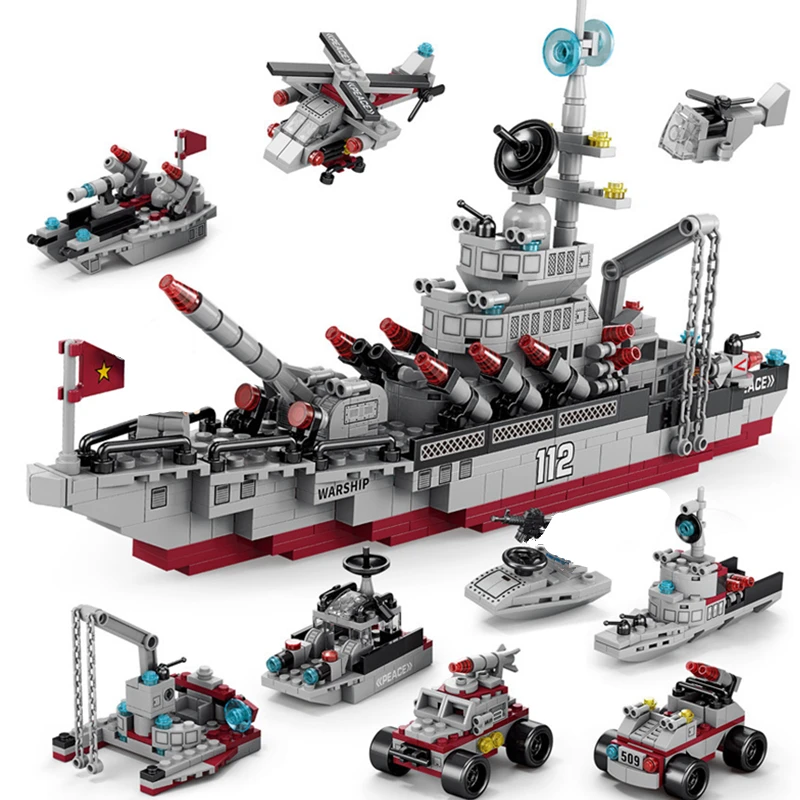The image, set against a white background, showcases a collection of intricately built military-themed Lego toys, presumably featured on the packaging of a Lego set. Dominating the center is a large, multicolored warship primarily in shades of red, gray, and black, accented with darker tones, and a hint of blue and yellow. This detailed warship bears the number "112" and the label "warship," and it’s outfitted with a red flag adorned with a yellow star. The ship is also equipped with multiple cannons and a prominent missile on top. Above the ship, a helicopter and a larger military-style helicopter hover, with an additional small helicopter on the top right of the image. The bottom of the image features six assorted vehicles, including two rover-like vehicles, a small speedboat, two additional ships, and machinery presumably designed for pulling the ships, which likely includes a tow truck. All items share a cohesive color palette, contributing to a unified and visually striking presentation of this comprehensive Lego set.